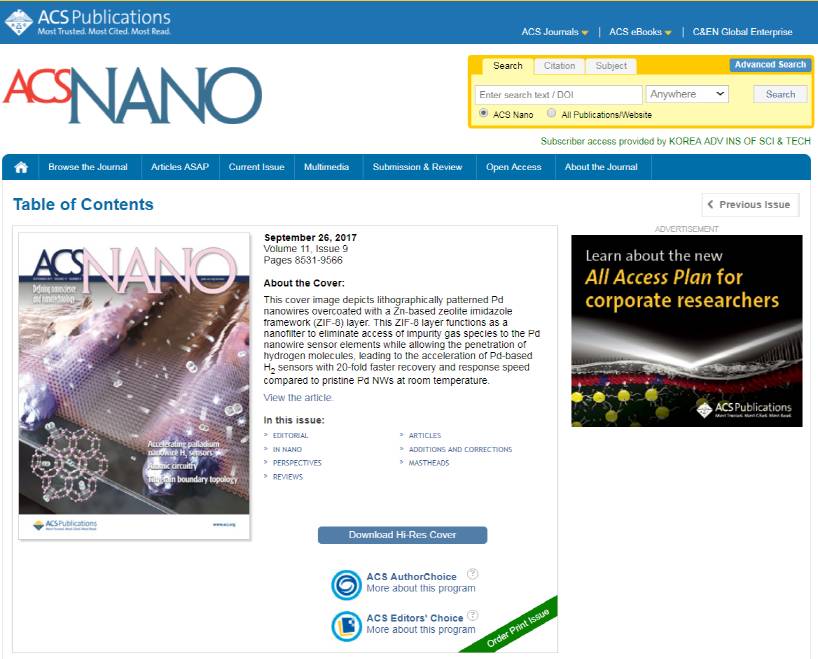This image appears to be a screenshot of a website, specifically under the category of academic resources. At the top, there's a prominent blue navigation bar displaying "ACS Publications," followed by the phrases "Most Trusted, Most Cited, Most Read." The same blue bar also includes links labeled "ACS Journals," "ACS eBooks," and "C&EN Global Enterprises."

Below this, there’s a white bar prominently featuring "ACS" in red letters and "Nano" in blue letters. Within this white bar, there’s a yellow search box offering options such as "Search," "Citation," "Subject," and "Advanced Search." Next to this, there's a text entry field for search queries along with a dropdown menu currently set to "Anywhere," allowing users to presumably select other specific areas for search. This search function also includes options to search within "ACS Nano" or across all publications on the website.

Further down, another blue bar hosts a comprehensive menu with options including "Browse the Journal," "Articles ASAP," "Current Issue," "Multimedia," "Submission and Review," "Open Access," and "About the Journal." Directly beneath this menu lies the table of contents, providing users easy navigation to various parts of the journal's content.